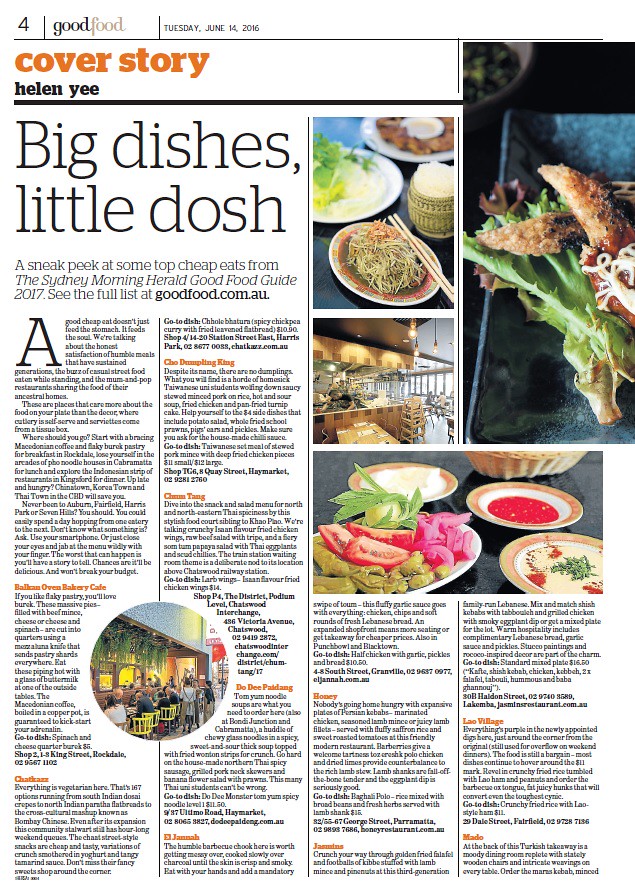In this captivating image, renowned food critic Helen Yee delves into a cover story featuring an array of delectable, budget-friendly dishes from the Sydney Morning Herald Good Food Guide 2017. The spread showcases a tantalizing selection of what are heralded as some of the best cheap eats in Sydney. These culinary gems are celebrated not just for filling the stomach, but for nourishing the soul with honest, satisfying meals that have stood the test of time. 

The photo encapsulates the vibrant buzz of casual street food, the humbleness of mom-and-pop restaurants, and the genuine care for food that transcends superficial decor. It portrays an authentic dining experience where diners fetch their own cutlery, and napkins are pulled from a tissue box, emphasizing a focus on taste and tradition over ambiance.

For a comprehensive list of these top affordable eateries, visit www.goodfood.com.au, where you can explore detailed food menus, enticing food items, and vivid images that bring this story to life. This guide is a celebration of the simple joys of eating, highlighting places where the food on your plate matters most.